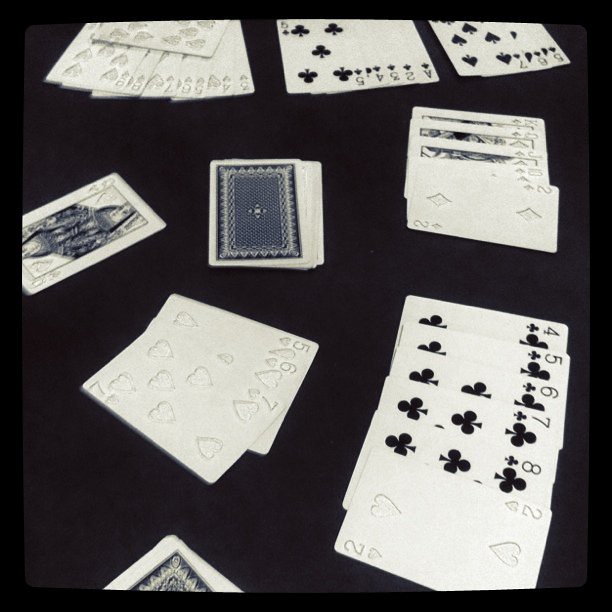The photograph showcases an organized array of black and white playing cards fanned out intricately on a black surface. In the bottom right corner, a hand of cards cascades in a fan shape, displaying sequential values of 2, 8, 7, 6, 5, and 4. A space separates this from another hand beginning with 2 and followed by 10, Jack, Queen, and King, all aligned in parallel straight lines.

At the top section of the image, three cards 5, 6, and 7 are positioned on the right-hand corner. The center section features a neat arrangement of Ace through 5. On the far left, a hand comprising cards 3, 4, 5, 6, 7, 8, and 9 is displayed, with one additional card overlapping the set.

A solitary Queen card lies on the left side of the table. Central to the photograph is a face-down deck of cards, positioned directly above a sequence of 5, 6, and 7. In the bottom left corner, the edges of a stack of face-down cards are visible. The majority of the cards clearly show black suits arranged in matching sequences, while several white cards have their suits indistinctly displayed.